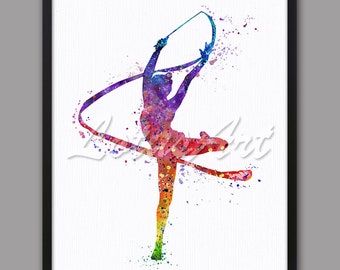The image features a wall-mounted artwork set against a gray background with vertical stripes on either side. The central focus is a white background showcasing a vibrant depiction of a ballerina or rhythmic gymnast. This figure is composed of rainbow-colored blotches, giving her an ethereal, watercolor-like appearance. With arms outstretched above her head, she gracefully holds a wand from which a long, multicolored ribbon flows and twirls around her, transitioning from blue near her hands to red and orange around her body, down to green near her planted foot. The ribbon creates a dynamic sense of motion. The artwork captures the essence of rhythmic dance and gymnastics, with the figure's fluid pose and the burst of colors enhancing the sense of movement and grace. This captivating image serves as a striking piece of decorative art.